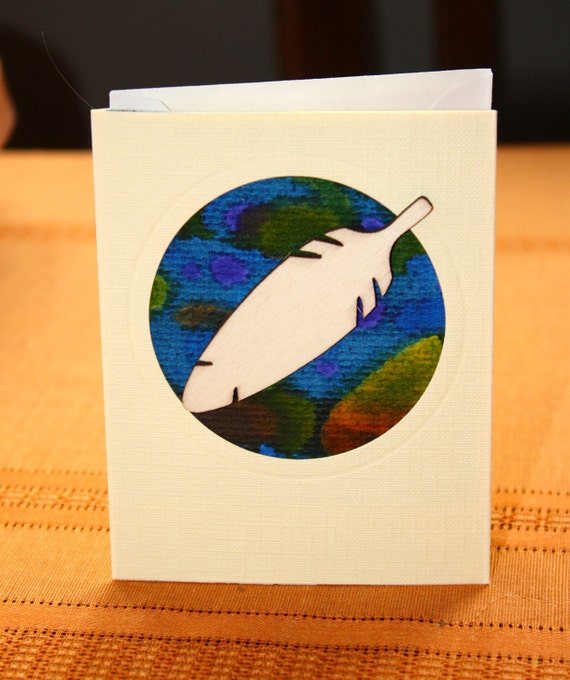The image features a greeting card standing upright on an orange tablecloth with subtle stitching on the edges, set against a blurred black background. The card itself is crafted from an ivory, textured cardstock and depicts a hand-drawn, watercolor-style illustration of the Earth. The Earth is rendered in a circular design prominently placed in the middle of the card, featuring blue, brown, green, and yellow hues, which create an organic and vibrant look. Centrally overlaying the Earth illustration is a vertically positioned white feather, intricately detailed, possibly as an applique that adds a three-dimensional aspect to the card. This elegant composition suggests it may be an Earth Day card, celebrating nature with its artful and symbolic design.